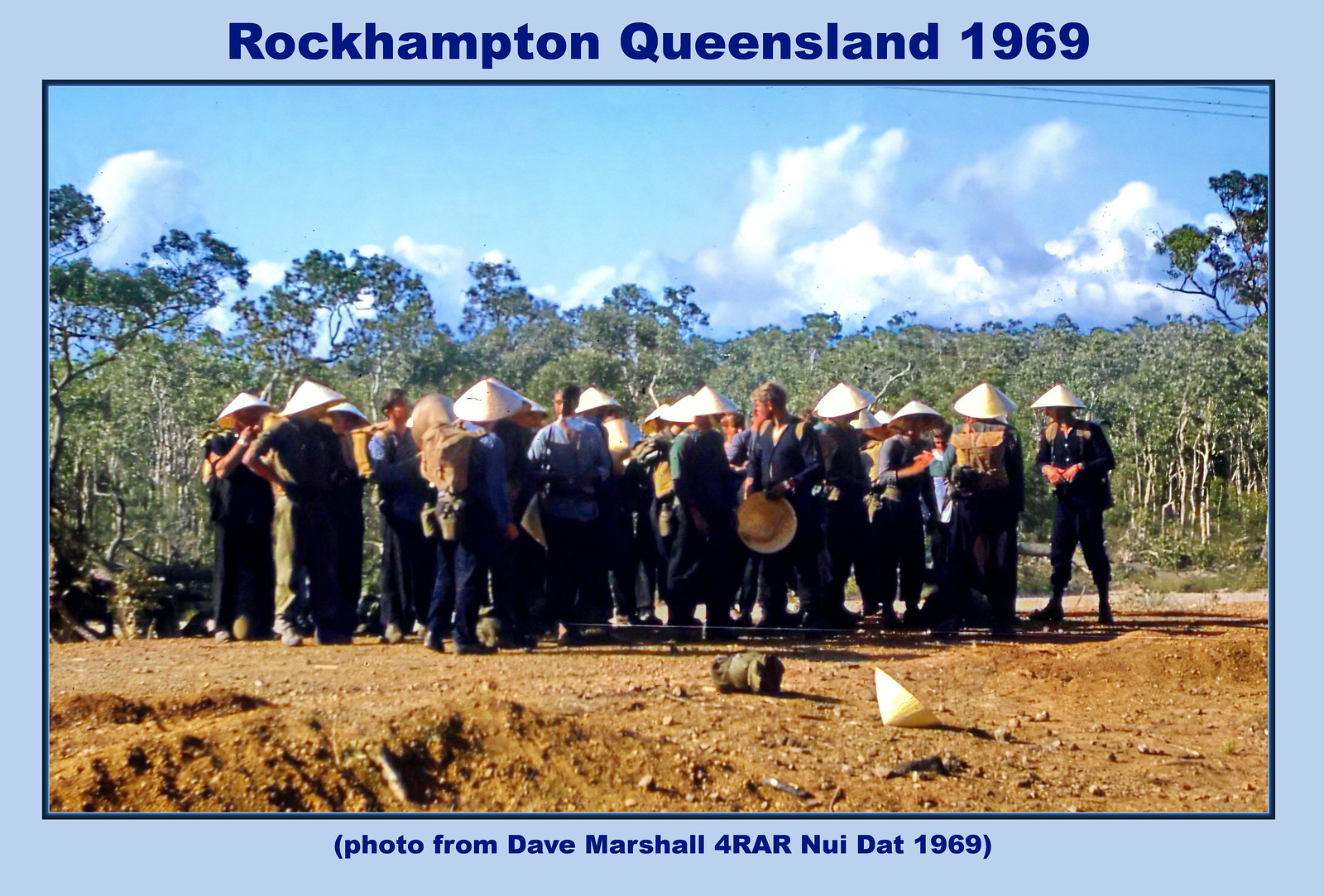This photograph, titled "Rockhampton, Queensland, 1969," sourced from Dave Marshall for 4RAR NUI DAT 1969, captures a group of approximately 20 people standing closely together on brown dirt ground. The individuals, predominantly dressed in dark clothing, with one in a blue shirt near the center, and another on the far right in a black suit with arms crossed, are wearing and holding straw-colored dome hats, with one hat and a green bag visible on the ground. Behind them is a dense row of trees with green leaves and white trunks. The sky above is a mix of blue and scattered clouds. The text "Rockhampton, Queensland 1969" with a light blue border around the top and sides and "photo from Dave Marshall for 4RAR NUI DAT 1969" underneath emphasizes the historical and locational context.